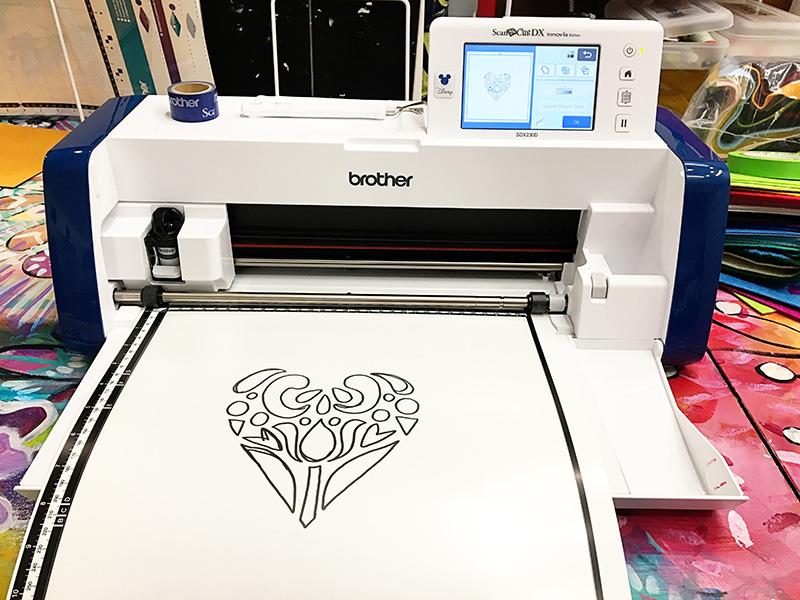The image depicts a Brother printer, specifically the ScanNCut DX model, prominently positioned on a vibrant, multicolored desk. The printer, a sleek, modern device in white with distinct blue trims, has "Brother" written in blue lowercase letters on its front. It features an LED screen displaying the illustration being printed—a black and white, heart-shaped design composed of various geometric shapes. The printer sits on a lively tablecloth adorned with shades of pink, blue, purple, and green, surrounded by colorful materials including printer paper, boxes of crayons or markers, and art supplies, indicating its use in a creative, art-focused environment. Additionally, there's a blue spool marked "Brother" placed on top of the printer, further emphasizing its brand and functionality in producing diverse designs. The sophisticated control panel with numerous buttons adds to its modern and versatile appeal.